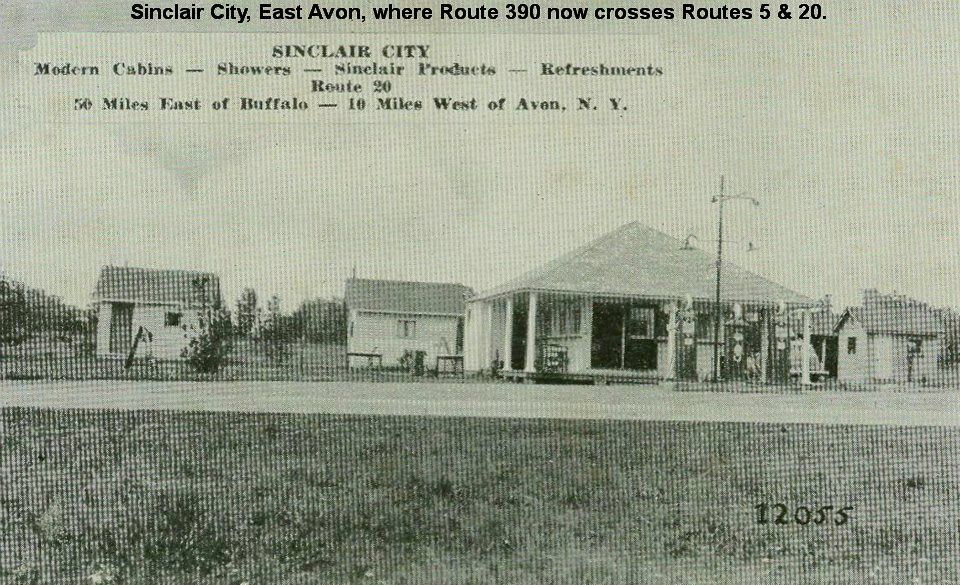This image, likely an old, black-and-white photograph or a photorealistic scan of a photograph, depicts a street scene with distinct pixelation suggesting an older printing technique. The image features a significant single-story building with a pointed roof, large doors, and windows situated towards the right side. Flanking it are smaller white-walled shacks, one on each side. A light-colored road spans from right to left across the scene, with a patch of textured ground in the foreground that appears to resemble grass or greenery. 

Overlay text at the top centered in what looks like digital print reads: "Sinclair City East Avon where Route 390 now crosses Routes 5 and 20." Additional printed text towards the top left says: "Sinclair City," followed underneath by "modern cabins, showers, Sinclair products, refreshments". It further specifies the location as being on Route 20, 50 miles east of Buffalo and 10 miles west of Avon, New York. The number "12055" is visible in the lower right-hand corner of the image.